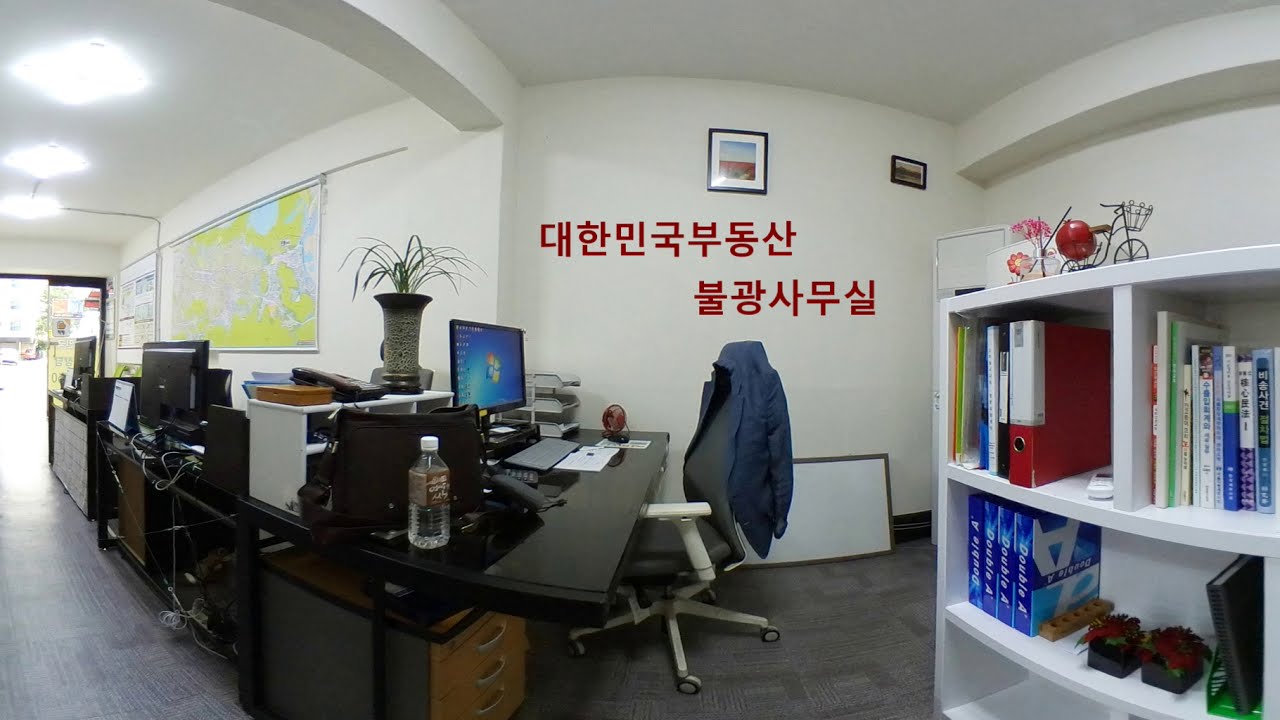The image depicts a modern office room, likely located in Korea suggested by the prominent Korean text in red letters on the white walls. Central to the room is a black laminate desk hosting a computer displaying the Windows logo, a white office chair with castered wheels, and a blue suit jacket draped over its back. To the right of the desk is a bookshelf with books that bear Korean text on their spines, along with a toy bicycle and a small red apple displayed on top. The room’s walls and ceiling are white, with the ceiling featuring recessed, elevated white lighting. On the left side of the room, a long black desk with multiple computers lines the wall, and a map hangs above it. A doorway on this side leads to a hallway, giving a sense of openness to the space. The office exudes a tidy and organized atmosphere, with clean surfaces and an array of neatly arranged office supplies and decorations.